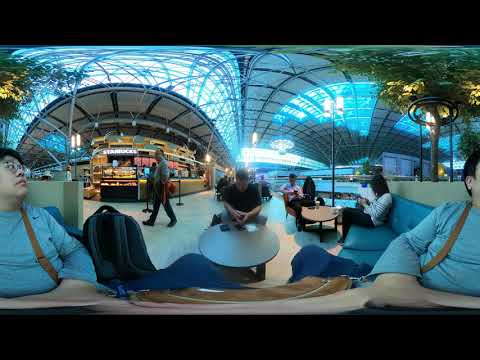The image depicts a brightly lit, indoor setting, possibly a shopping mall or food court, characterized by a panoramic shot that seems to merge two separate images into one wide view. At the center stands a small round table, where a Caucasian man with short hair leans over, seemingly engrossed in his phone. Surrounding him, a scene unfolds with people sitting and relaxing. In the foreground on both the left and right sides, there is an Asian woman with dark hair and clear glasses. She is dressed in a gray shirt and has a strap, possibly from a purse or backpack, slung over her shoulder. This woman is seated in a blue leather-padded area, and her image appears to be repeated, adding to the panoramic effect. The background features a curved structure with numerous shops, including what seems to be a Starbucks, and is supplemented by benches occupied by other individuals. Elements such as fake trees and a large glass ceiling that allows ample light to enter suggest an open, spacious indoor environment. The image is bordered by black at the top and bottom, with a mix of colors present, including black, brown, light blue, gray, yellow, green, pink, tan, dark blue, and white, providing a vibrant and busy ambiance.